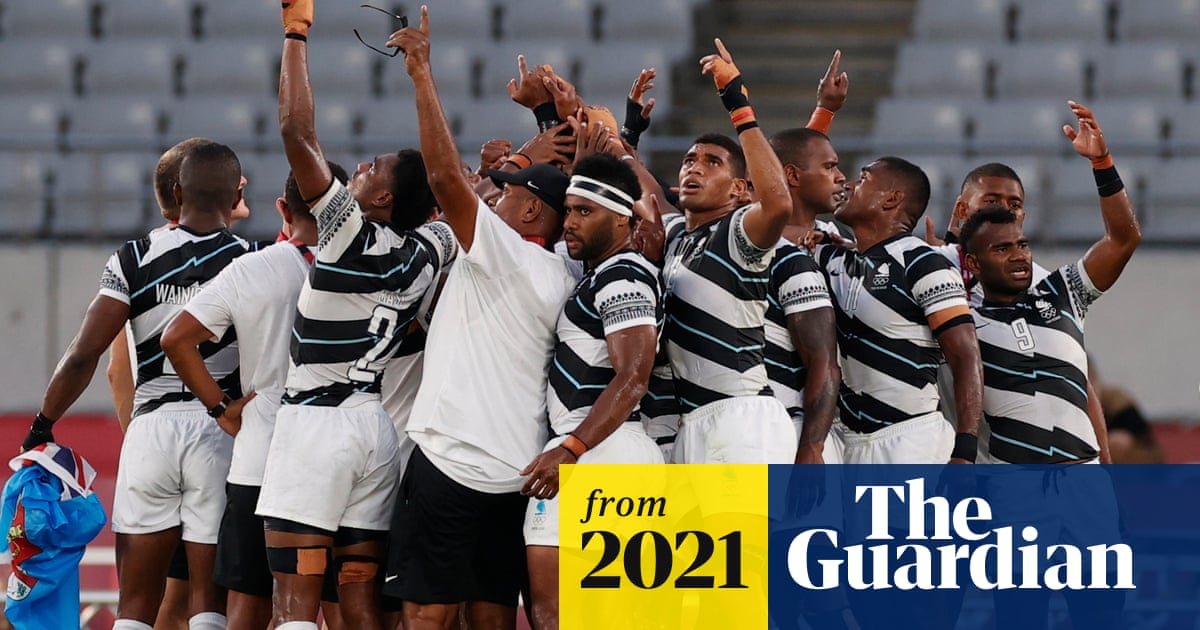This detailed caption consolidates the various descriptive elements provided:

---

This is a photograph of a sports team, likely soccer, celebrating or gearing up for an event in an empty stadium with gray bleachers in the background. The team consists predominantly of dark-skinned men, suggesting a mix of African, Latino, and potentially Indian players. They are shown wearing uniforms that feature white shorts and shirts with black and light blue diagonal stripes, or in some cases, white shirts paired with black shorts. One man in the foreground stands out with an orange and black glove on his left hand, fingers exposed, looking up with a serious expression. The players are all raising one arm toward the sky, and their expressions range from serious to shocked. At the bottom right corner of the image, a banner is split into two sections: the yellow section reads "From 2021" in black text, and the blue section reads "The Guardian" in white text. Additionally, there is a visible red clay track behind the players, contributing to the stadium setting.